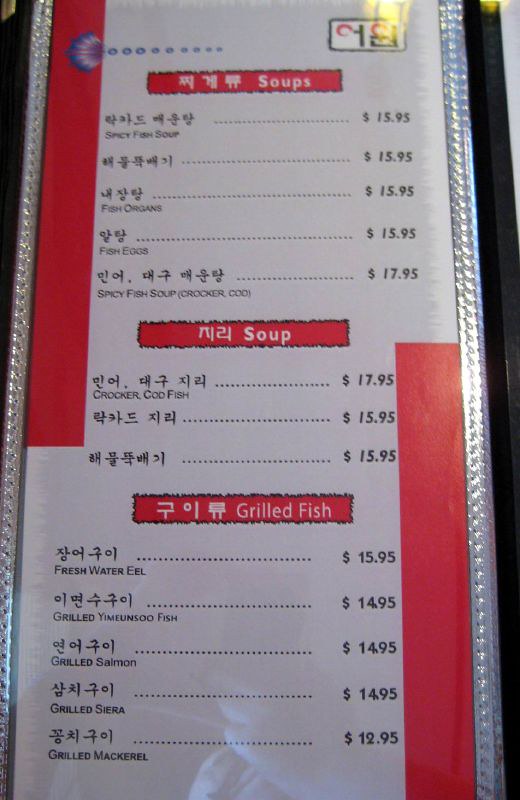The image depicts a menu displayed outside a dining area, framed by vertical metal bars on either side. The menu is illuminated by yellow lighting with its surface reflecting the light. Text on the menu is predominantly in Japanese, Korean, and Chinese characters with English translations for many items, though some remain untranslated. The items are categorized into three main groups: "Soup," "Soup (Singular)," and "Grilled Fish." The menu features blocks of red in both the lower right and upper left corners. In the upper left, there is an intricate symbol resembling a shell, composed of concentric circles in shades of purple, pink, white, and hints of red. Prices are marked with dollar signs, with items priced in two-digit figures to the left of the decimal point.